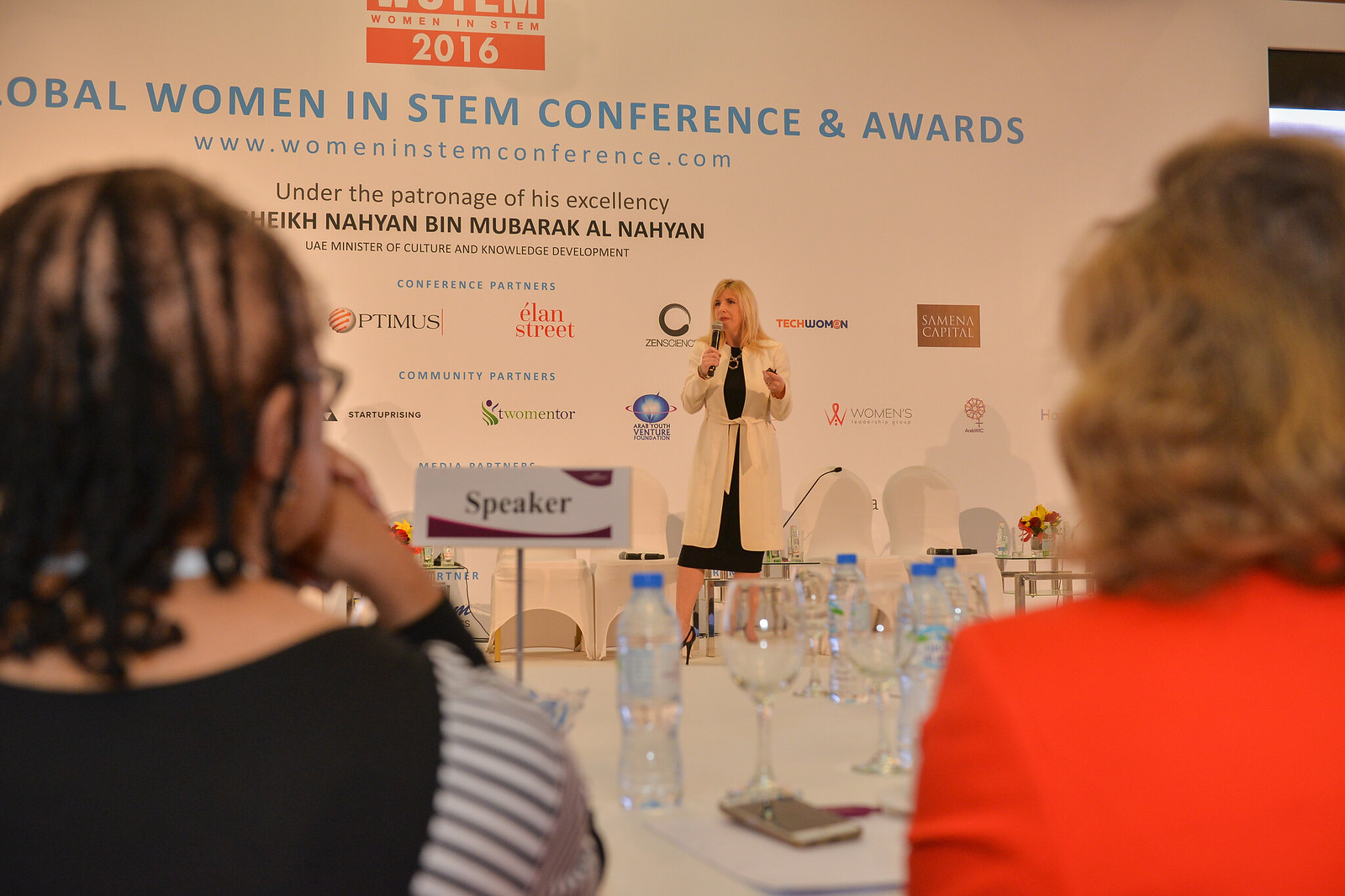The image captures a moment from the 2016 Global Women in STEM Conference and Awards, held under the patronage of His Excellency Sheikh Nahyan bin Mubarak Al Nahyan, the UAE Minister of Culture and Knowledge Development. On stage, a woman stands confidently, clad in a white jacket over a red and black dress, holding a black microphone. The backdrop prominently displays the event title and the website, www.womeninstemconference.com, along with various sponsors including Optimist, Elan Street, Tech Women, Semitic Capital, and Star Uprising.

In the foreground, two women are seated at a table. One is wearing a black dress with white accents on the sleeves, while the other is in a red dress, her cellphone placed nearby. The table is set with water bottles, champagne glasses, and a placard that reads "Speaker." The scene reflects a professional and empowering atmosphere, celebrating women's achievements in STEM.